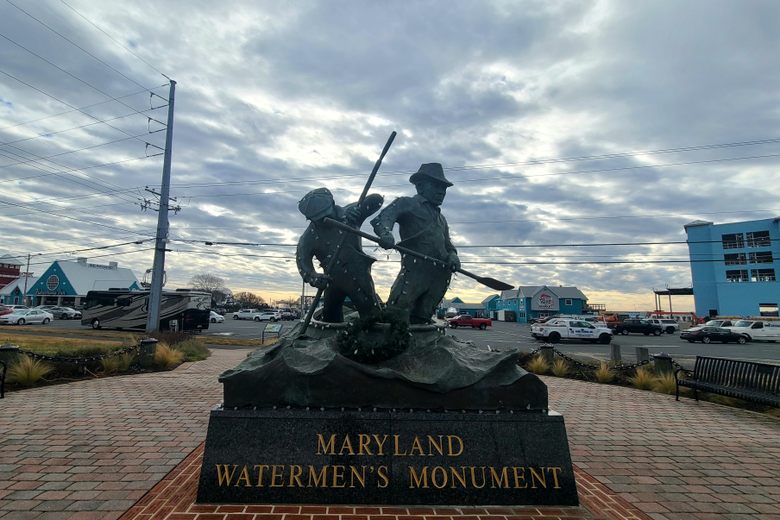This photograph, taken outdoors on a gray, cloudy day, showcases the Maryland Watermen's Monument prominently displayed on a brick walkway. The majority of the bricks are a faded red, but the statue sits on a section of darker red brick. The dark gray statue depicts two men in a rowboat, each holding an oar and wearing hats, navigating through rough waters intricately carved at the base. The solid black cement base of the monument features the inscription "Maryland Watermen's Monument" in gold lettering. Surrounding the statue, on the right, is a metal black bench, while a telephone pole with numerous wires appears to the left. The background reveals a mix of parked cars and trucks, a blue parking garage, and several stores and houses. The overall scene suggests it is part of a park courtyard or similar area, with hints of restaurants nearby. Additionally, the monument is adorned with Christmas lights, adding a touch of seasonal decor.